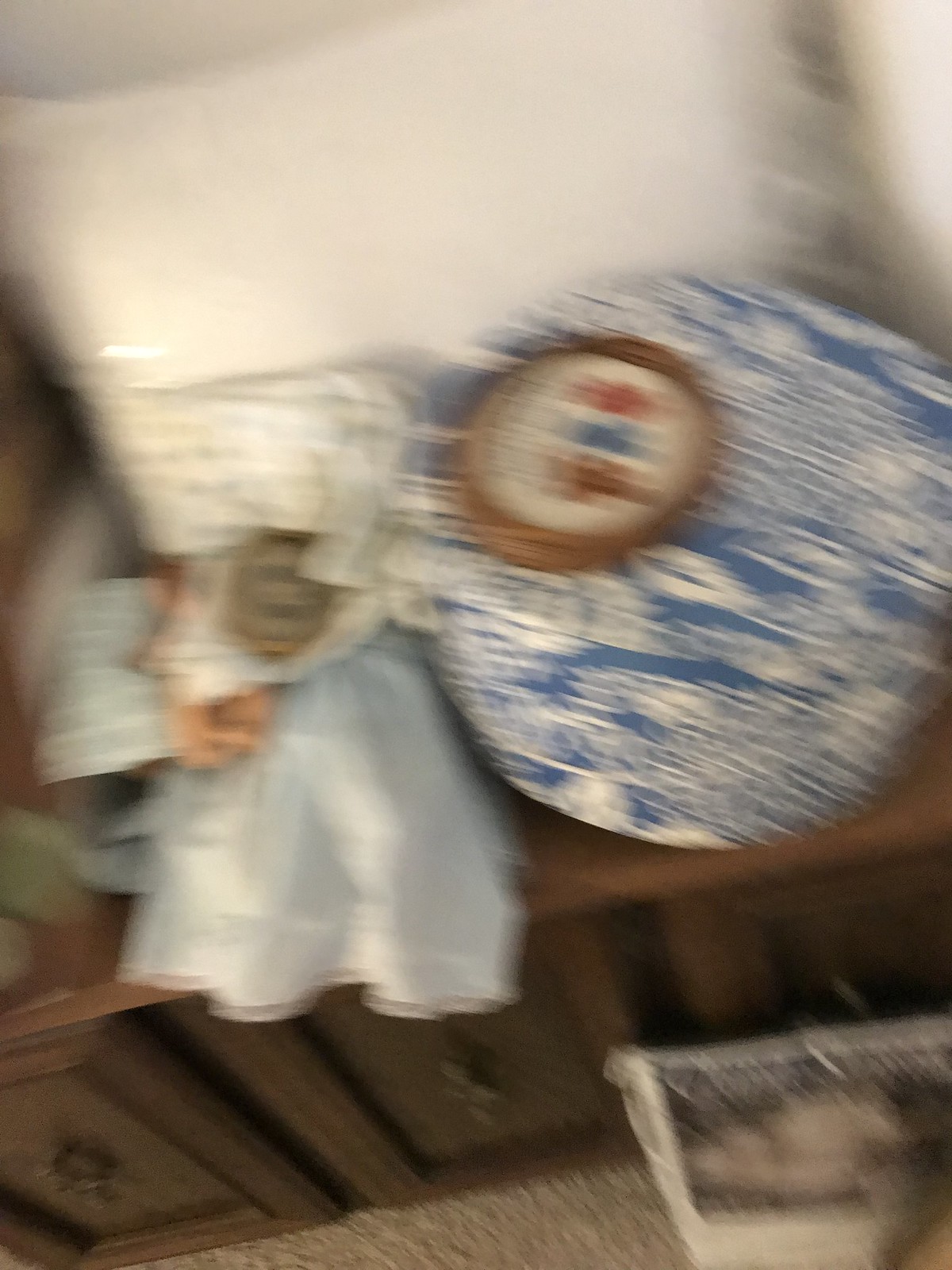A somewhat blurry image depicts a dark brown dresser with elegant, ornate metal handles, possibly brass. On top of the dresser, various items are arranged. To the right, there is a circular blue and white box adorned with a floral, leaf-like pattern. Above the box sits an embroidery hoop with a medium wood frame featuring an intricate design incorporating brown, blue, and red shapes set against a white background. Also visible on top of the dresser is a pile of clothing, including a white christening gown and a mixture of beige and orange fabrics, which might be part of sewing or embroidery projects. Behind these items rests a large rectangular white pillow. In the lower right corner of the image, near the dresser, is a white or clear bag, possibly a shoe bag, resting on the floor. The white wall in the background frames the scene, and a carpeted floor is discernible beneath the dresser.